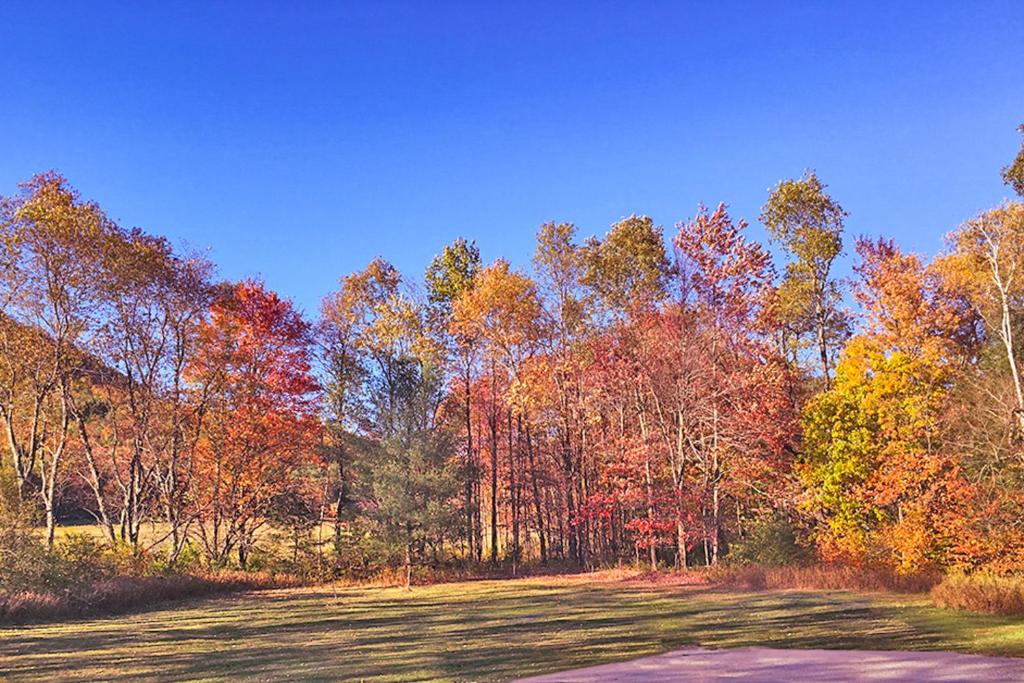The image captures a picturesque fall scene featuring a beautiful mixture of vibrant autumn colors against a clear, azure blue sky. In the foreground, a gray concrete pad is partially visible on the lower right, bordered by a lush expanse of green grass that is cast with shadows from the trees above. The middle ground is dominated by a variety of trees showcasing a stunning array of leaf colors, including greens, reds, browns, yellows, and oranges. These trees, which appear to include birches and possibly walnuts, form a dense line that creates a natural-looking barrier. Scattered leaves on the ground emphasize the season. Behind this vibrant tree line, there's an open field and distant mountains partially obscured by the foliage, suggesting a serene and tranquil landscape. With the sky being a clear and vivid shade of blue, and the overall stillness of the leaves indicating minimal wind, the scene likely typifies a crisp fall day with mild temperatures, evoking the essence of late September or October.